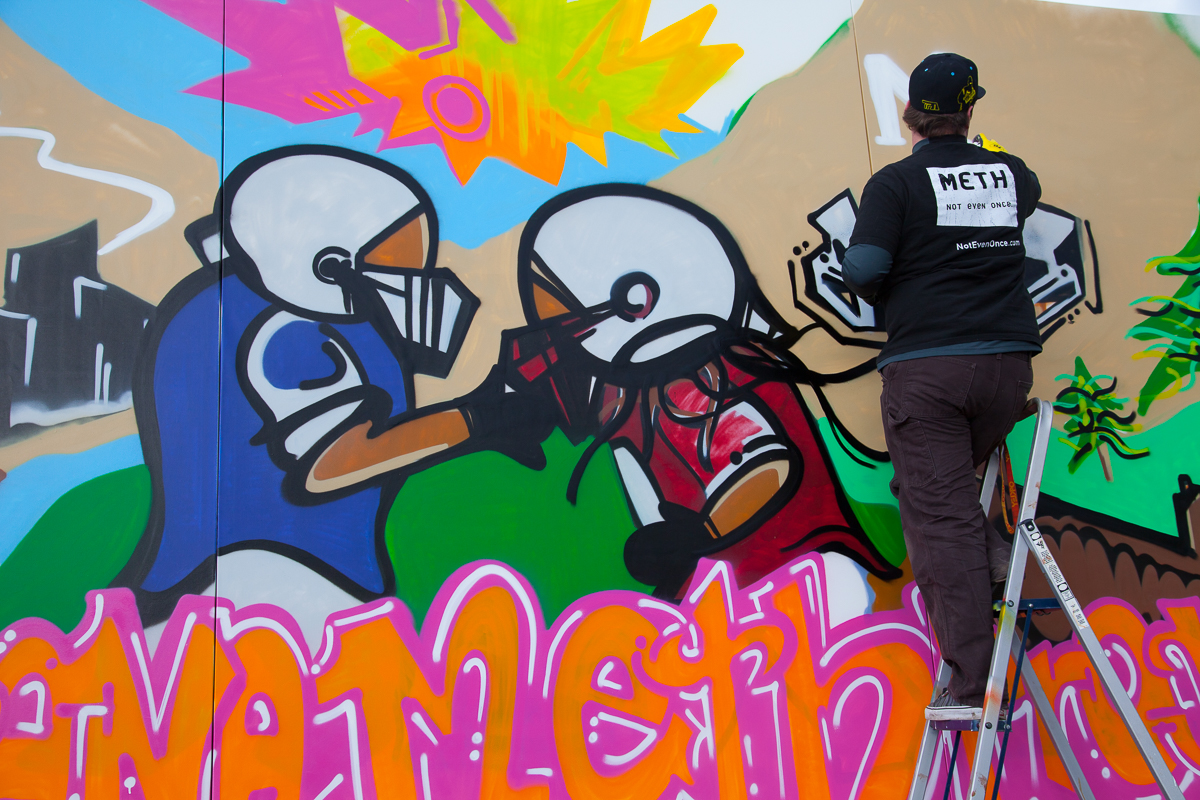An outdoor color photograph shows a man on a tall, silver ladder, his back turned to the camera, painting a mural on the side of a building. He is a fairly large individual, dressed in brown pants and a green shirt, with a green baseball cap on his head. The back of his shirt displays a white rectangle with blue letters spelling out "METH." The majority of the image is dominated by the mural he is working on. The mural features two cartoon-styled football players, visible from the waist up and depicted in profile, as though they are facing each other. Both players wear white helmets; the player on the right, in a red jersey, appears to have their elbow bent as they touch the face of the player on the left, who is dressed in blue. The scene is rich with vibrant colors, including green waves and trees on the right, a blue blob interspersed with pink, yellow, and green toward the top, and some undecipherable orange lettering at the bottom. Despite disparities in clothing descriptions provided, it is evident that the man is actively adding his own touches to the mural, rather than erasing it.